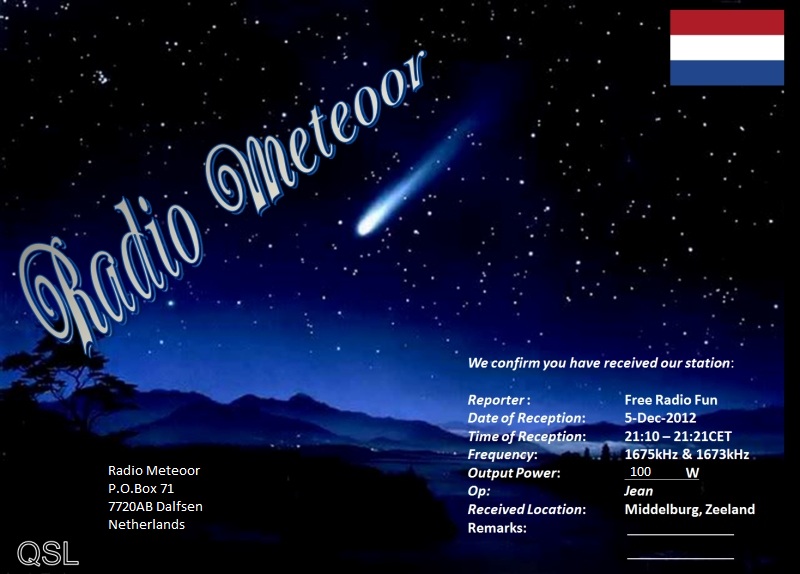The image resembles a PowerPoint slide with a backdrop depicting a night sky filled with white stars against a gradient of black and dark blue hues. The landscape at the bottom is composed of silhouettes of mountains and a tree in the bottom left corner. Diagonally, from the left-center of the image towards the top-center, the text "Radio Meteor" appears in white. In the top-right corner, there's a tricolor flag with horizontal red, white, and blue stripes. The bottom right corner contains multiple lines of text: "We confirm you have received our station. Reporter: Free Radio Fund. Date of reception: 5 December 2012. Time of reception: 2110 to 2121 CET. Frequency: 1675 kHz and 1673 kHz. Output power: 100 watts. OP: Gene. Receive location: Middelburg, Zeeland." Additional information includes a P.O. box address in the Netherlands in the bottom left corner, alongside the acronym "QSL."